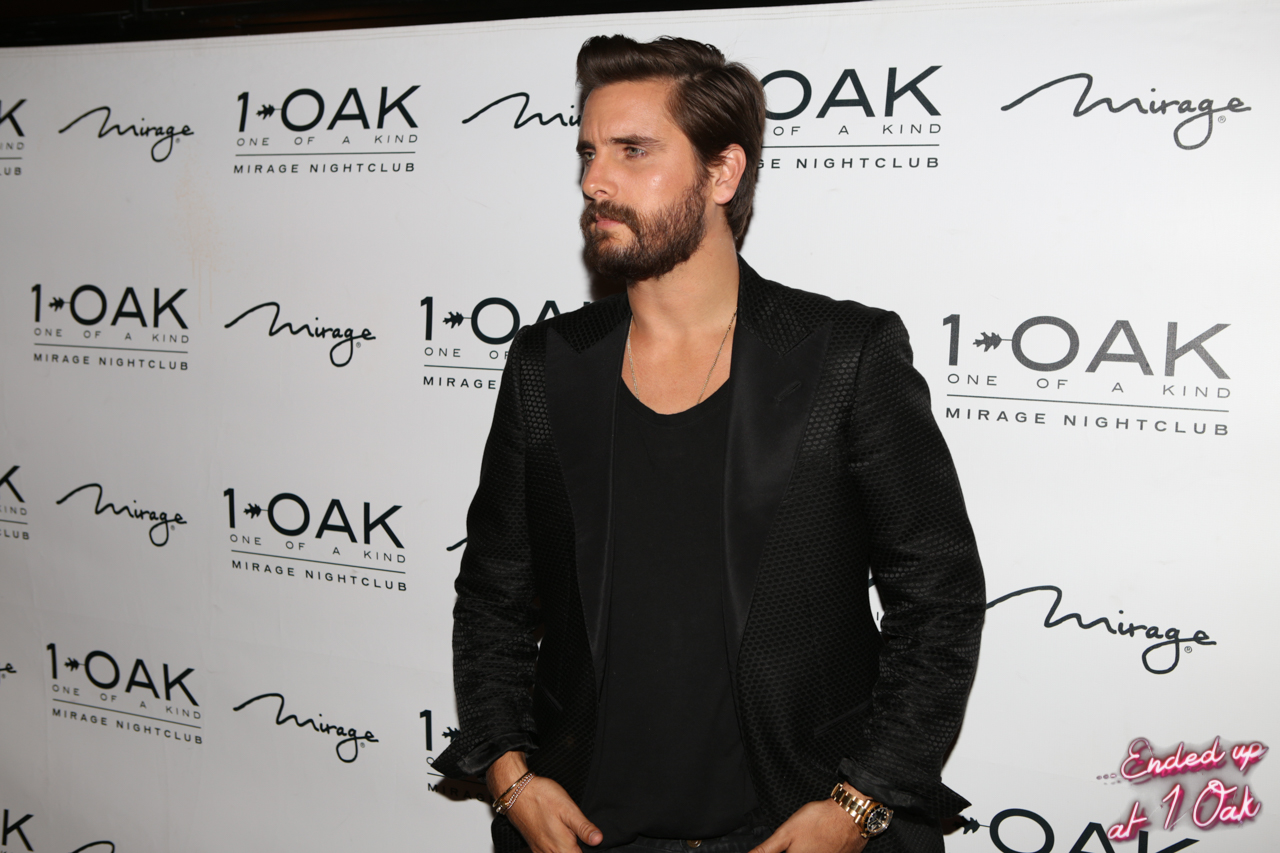The image captures Scott Disick at a press event, likely held at a nightclub, standing in front of a white backdrop adorned with a repeating pattern of logos, including "One Oak" (stylized as O-A-K with "One Of A Kind" beneath it), "Mirage Nightclub," and "Mirage." In the lower-right corner of the backdrop, pink and white text reads, "Ended Up at One Oak." Scott is dressed in a black t-shirt paired with a long-sleeved designer jacket, which appears to have a satin, snakeskin-like texture. His hair is meticulously groomed, slightly balding, slicked back, and he has a well-maintained brown beard. He sports a wristwatch on his left wrist and wears a stern, neutral expression while looking off to his right.